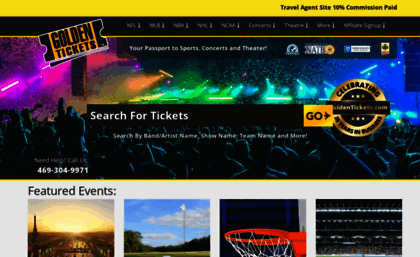The screenshot captures a ticket purchasing site, seemingly for concerts. At the top left, the logo "GOLDEN TICKETS" stands prominent with "GOLDEN" in all caps and larger font, while "TICKETS" is in slightly smaller caps. Across the top right, a yellow banner features the text "TRAVEL AGENTS SITE 10% COMMISSION PAID" in black. Below this banner, a black navigation bar lists various site categories from left to right: NFL, MLB, NBA, NHL, NCAA, CONCERTS, THEATER, MORE, and AFFILIATE SIGN UP. 

Beneath the navigation bar, the tagline "YOUR PASSPORT TO SPORTS, CONCERTS, AND THEATER" is visible, accompanied by several logos. In the page's center, there's a search field labeled "SEARCH FOR TICKETS," where users can enter their desired event, followed by a distinctive golden "GO" button to initiate the search.

Additionally, contact details are provided at the bottom left with the help number: 469-304-9971. The very bottom of the page hints at "FEATURED EVENTS," but the details are cut off and not fully visible in the image.